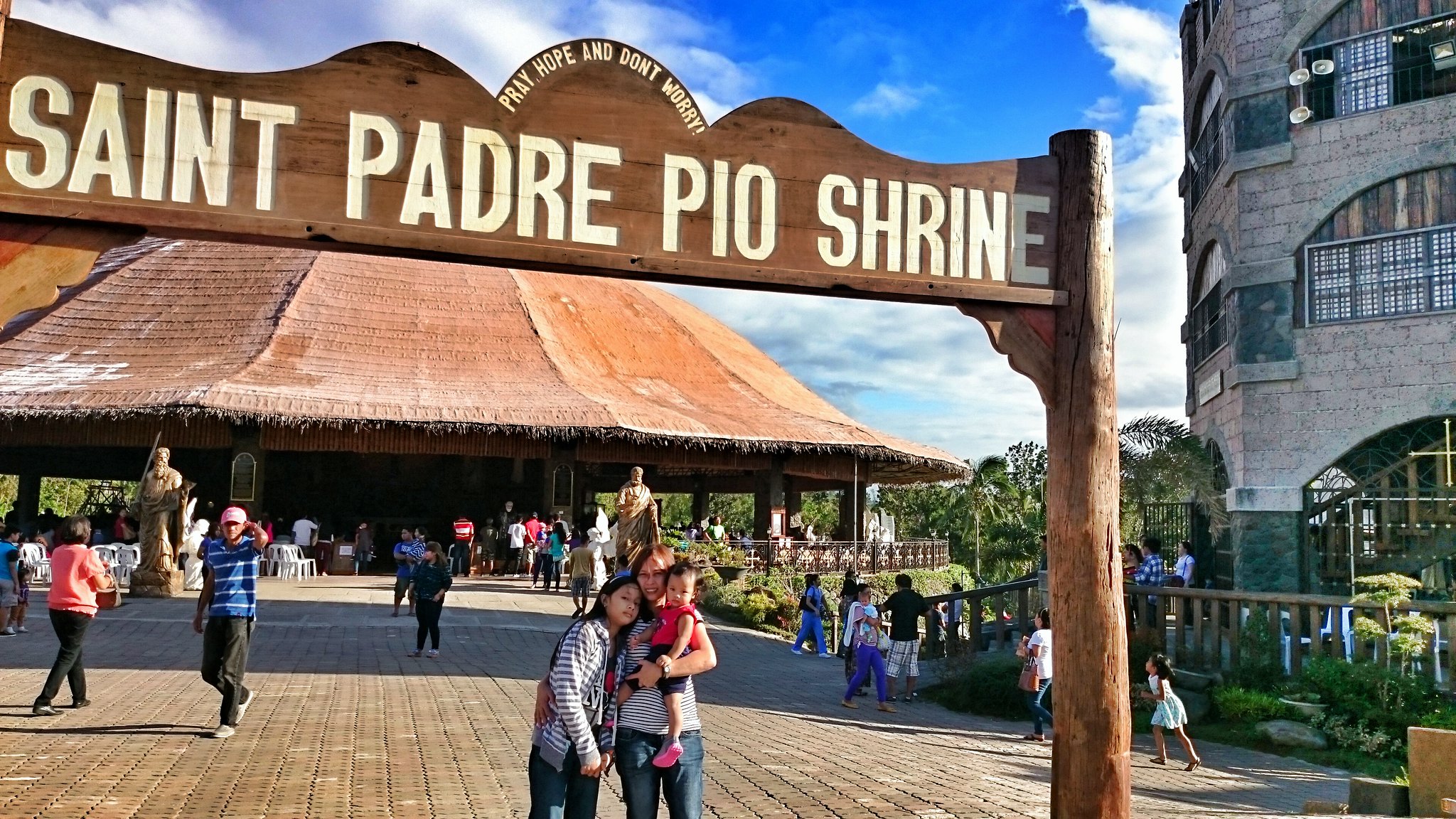In a bright daytime outdoor setting, a photograph captures a lively scene at the St. Padre Pio Shrine, with a vibrant light blue sky and occasional cloud cover above. The central focus features a woman posing with two girls, standing beneath a sign that reads, "St. Padre Pio Shrine. Pray, hope, and don't worry." The woman and the older girl are both dressed in stripes and jeans, while the younger girl sports a red shirt, black shorts, and pink sneakers. She is also holding a baby in her left arm.

The family stands on a stone brick walkway leading to a large courtyard framed by statues flanking either side. People can be seen walking to and from a covered terrace area resembling a large food court or seating area, with white plastic chairs scattered underneath. Buildings with stained glass windows and spotlights, along with lush trees, enhance the background scenery. The photograph is filled with bustling activity, including numerous visitors exploring the shrine and enjoying the day.